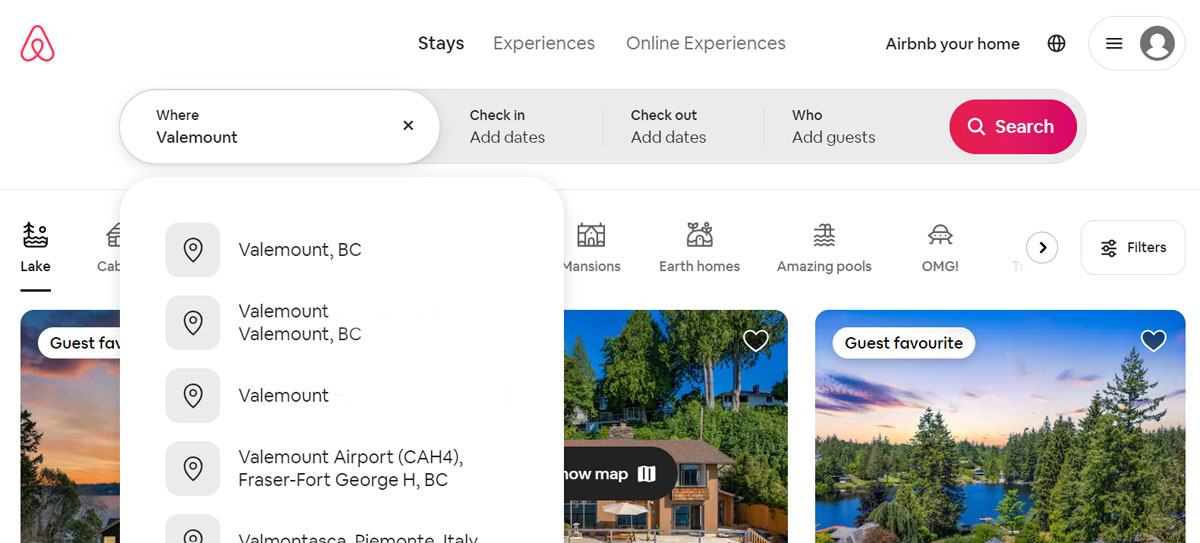This screen capture from the Airbnb website showcases the interface and search functionalities for finding accommodations. In the upper left corner, the Airbnb logo is prominently displayed. The top navigation bar includes options for "Stays," "Experiences," "Online Experiences," "Airbnb Your Home," and a log-in icon located on the far right. The "Stays" tab is currently selected, indicating the user is searching for places to stay.

Below the navigation bar is a search interface divided into several fields: "Where" with "Valmont" selected, "Check-in" and "Check-out" fields prompting the user to "Add Dates," a "Who" field to "Add Guests," and a "Search" button on the far right. When the "Where" field is expanded, a drop-down menu appears listing multiple location options such as "Valmont, BC," "Valmont Airport, CAH4," and "Fraser Fort George, HBC," among others.

Behind this overlay, the main section of the webpage is partially visible, with images of various Airbnb listings. The only clearly visible image to the right depicts a scenic lake, possibly in Canada, and is labeled "Guest Favorite." The overlay somewhat obscures the other images and details of the listings on the main page.